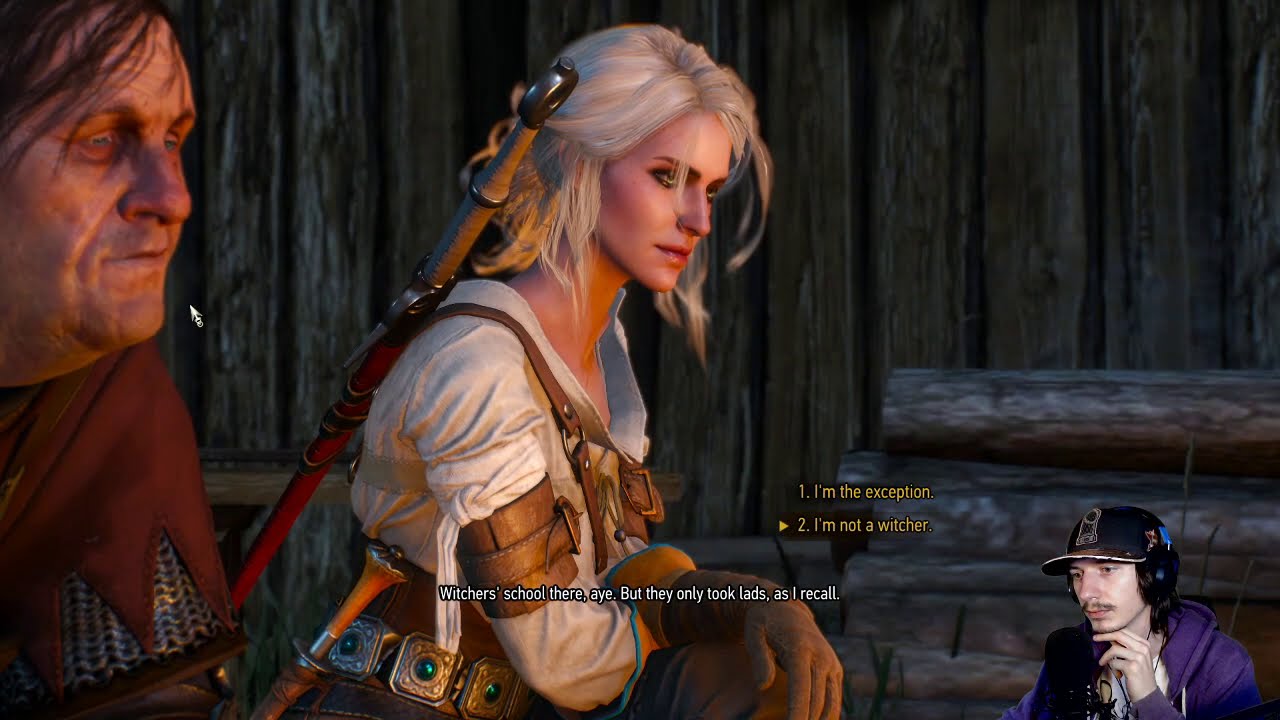The image is a screenshot of a streamer playing "The Witcher" video game. In the lower right-hand corner, there's a small video overlay of the streamer, who is wearing a black cap with a yellow rim, a purple sweatshirt, and a headset. The streamer, who has a brown mustache, is captured in a thoughtful pose with two fingers under his chin. To the left and center of the screen, the game displays two characters: an older, worn-out-looking man with straggly brown hair and maroon clothing, and a younger woman with white-blonde hair. The woman is dressed in medieval-style attire with various leather attachments and gloves, and she has a sword strapped across her back. The background of the game's scene features a wooden fence and a pile of wood. On-screen text offers dialogue choices: "I'm the exception" and "I'm not a Witcher," with additional text mentioning the Witcher School only taking lads. The streamer appears to be in the process of deciding how to respond in the game.